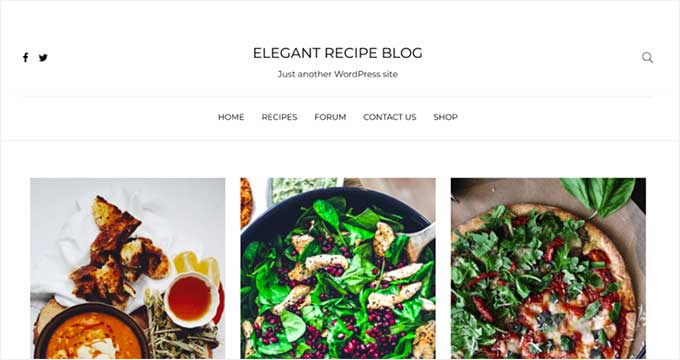This image is a screenshot from an elegant recipe blog. On the left side of the header, there are clickable icons for Facebook and Twitter. To the right, there is a clickable magnifying glass icon. Below the header, in smaller text, it reads "Just another WordPress site."

A series of faint gray lines divides the page into sections. The first section contains the navigation menu with the items "HOME," "RECIPES," "FORUM," "CONTACT US," and "SHOP," all written in bold, uppercase black letters against a white background and evenly spaced.

The next section, also divided by a faint gray line, showcases three images. The left image features a serving of curved toasted bread beside a bowl of tomato soup paired with a small dipping sauce. The center image displays a fresh salad topped with chicken strips. The right image shows a homemade pizza garnished with spinach, different herbs, and olives.